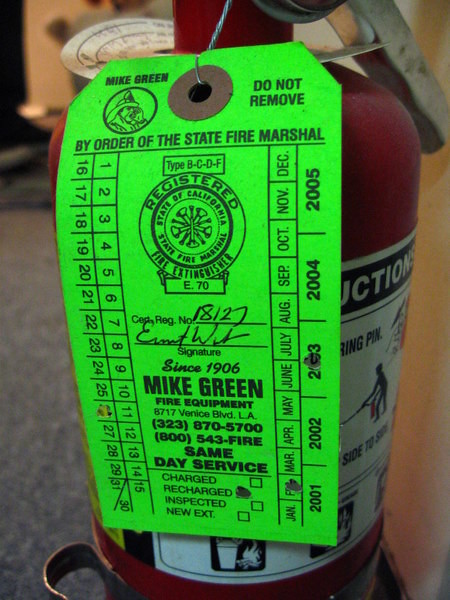This image is an extreme close-up of a bright green inspection tag attached to a red fire extinguisher, set against a background that appears to be gray carpeting. The tag prominently features the name "Mike Green" in the upper left corner, alongside an emblem labeled "State of California, State Fire Marshal, Registered Fire Extinguisher." Below, it includes the certification number "CED Reg number 18127" and contact details: "Mike Green Fire Equipment, 8717 Venice Blvd, LA, 323-870-5700 or 800-543-FIRE, same-day service." The top right of the tag sternly states "DO NOT REMOVE" in black capital letters, followed by "By Order of the Fire Marshal."

The tag is highly detailed, showing inspection information with punched marks indicating key dates: "26th" under the days, "February" under the months, and "2003" under the years. The bottom section contains checkboxes for "Charged," "Recharged," "Inspected," and "New EXT," with "Recharged" being filled in. The tag emphasizes the importance of the fire extinguisher's maintenance history, critical for safety adherence.